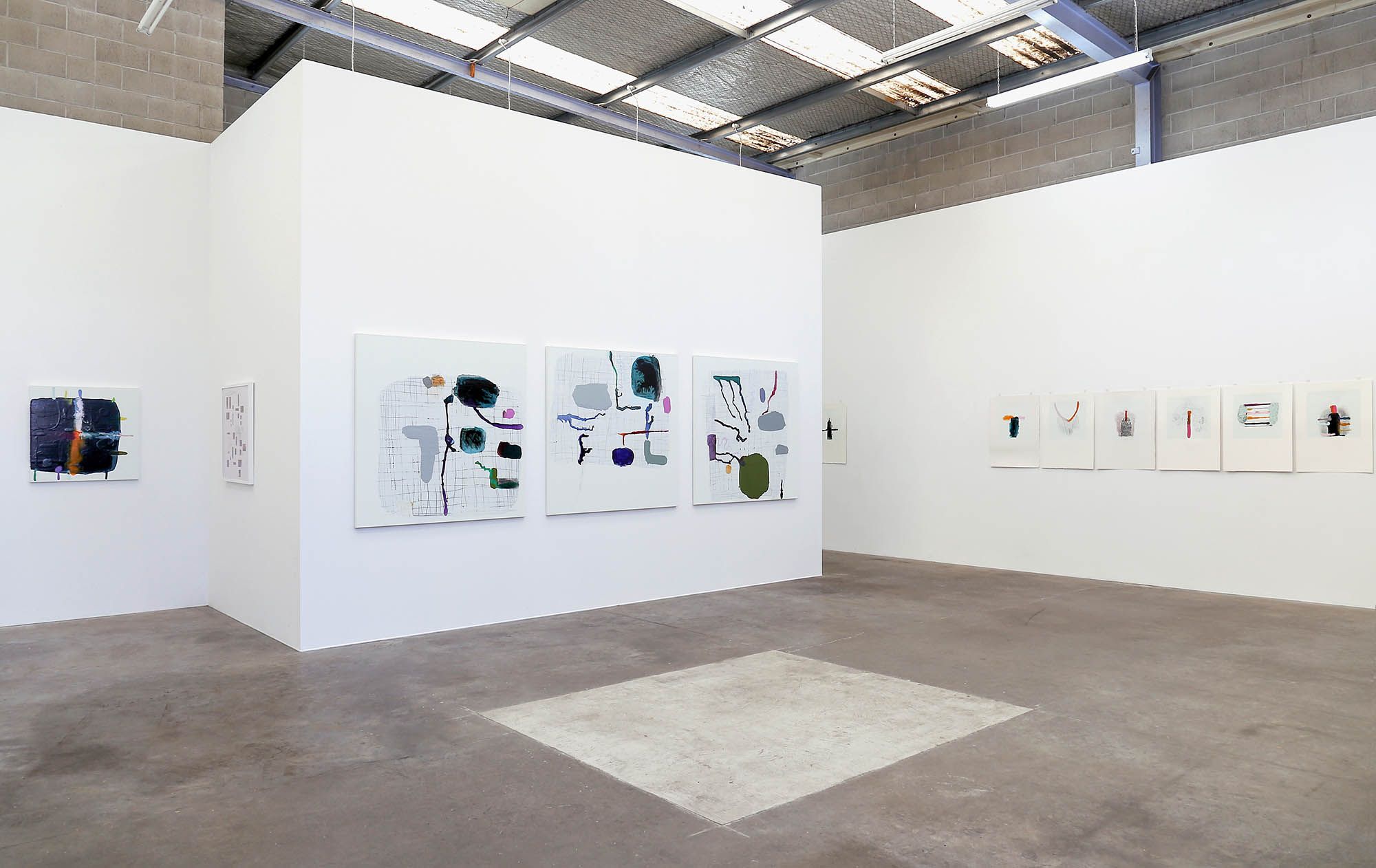The image depicts a modern art gallery set in a converted warehouse with distinct industrial elements. The setting features polished gray concrete floors and white walls that are juxtaposed against gray cinder block walls higher up, near the corrugated steel ceiling, which incorporates clear plastic panels for light. The gallery space includes a notable white protruding wall that showcases three large, abstract, and minimalist paintings. These paintings feature white backgrounds adorned with rectangular and oval gray splotches, interconnected by red and gray lines, squiggly details, and cloud shapes. A glowing white rectangle is strategically placed on the floor in front of this wall. To the right, another white wall displays six smaller abstract paintings, each maintaining the same minimalist aesthetic with themes of gray rectangles, red lines, and cloud forms. Additionally, a corner wall behind the initial trio of paintings hosts another gray and white artwork, and nearby, a final painting features a striking black rectangle with red and blue L-shaped elements. The gallery is lit by fluorescent lighting, enhancing the contemporary ambiance of the space.